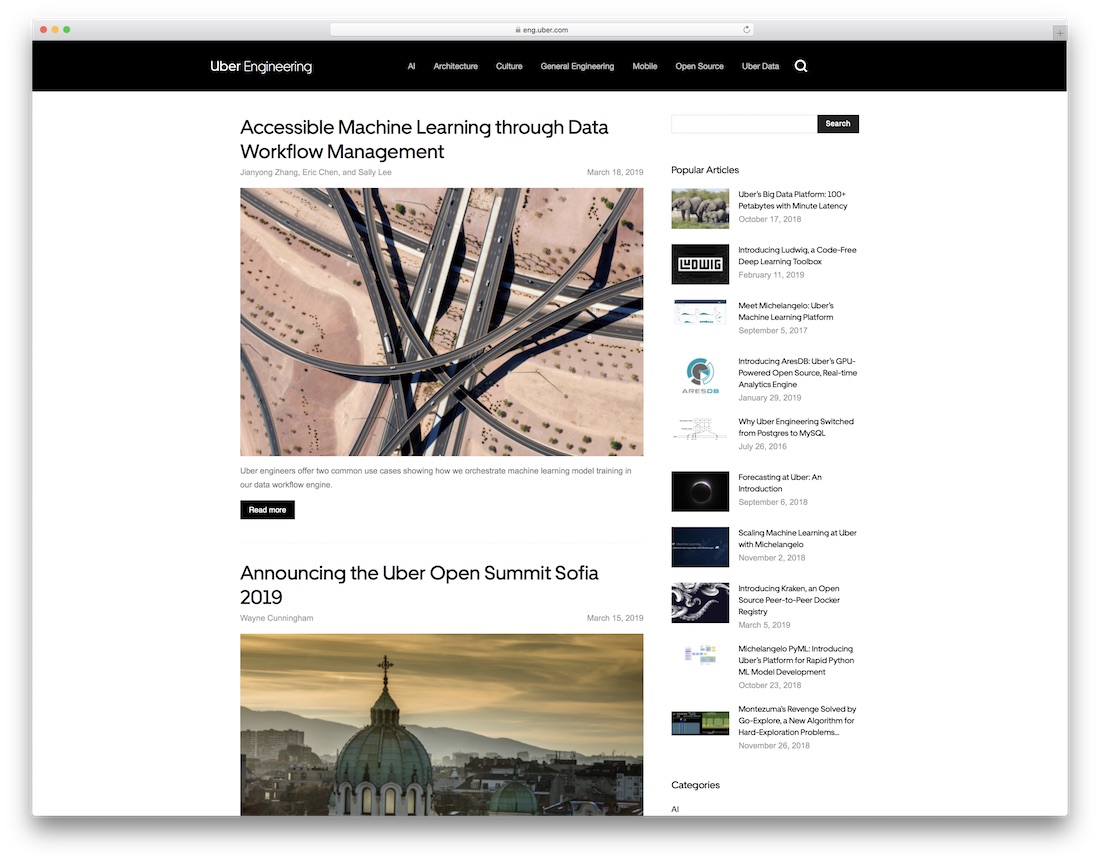A detailed and descriptive caption for the image could be:

"This horizontal screenshot, set against a white background with a misty gray shadowed border on its left, right, and bottom sides, features a webpage with a thin gray address bar at the top. Below it, a black banner bearing the title 'Uber Engineering' is flanked by links labeled AI, Architecture, Culture, General Engineering, Mobile, Open Source, Uber Data, and an icon of a magnifying glass for search functionality. The main content showcases two highlighted articles. The first article, featuring an aerial view of a complex highway interchange, is titled 'Accessible Machine Learning through Data Workflow Management.' The second article, marked by an image of a cityscape under a yellow and gray sky, is introduced with the heading 'Announcing the Uber Open Summit Sophia 2019.' On the right-hand side of the page, a vertical column contains a list labeled 'Popular Articles,' showcasing clickable links to different articles. At the top of this column, there's a search bar accompanied by a black search button."